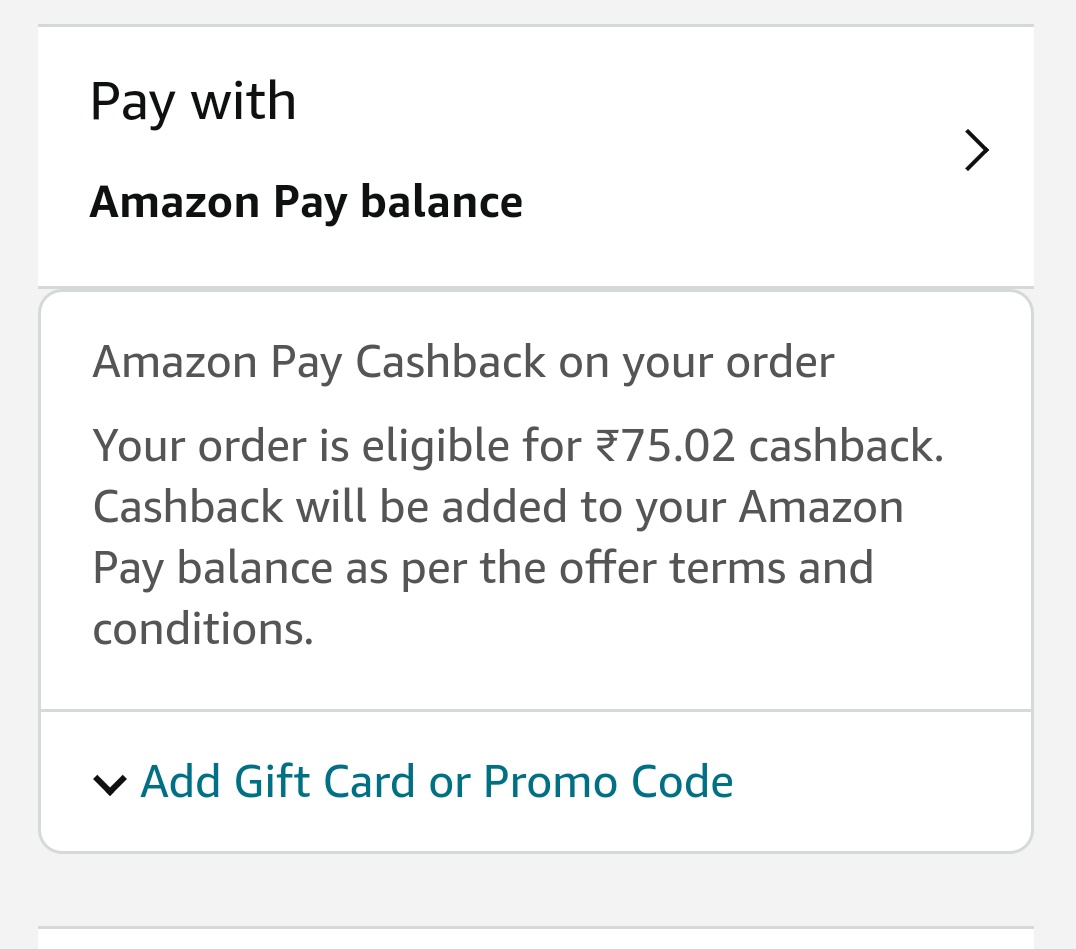The image shows a message indicating that the user can "Pay with Amazon Pay Balance," with a right-pointing arrow next to it. The text mentions that the order is eligible for a $75.02 cashback, which will be credited to the user's Amazon Pay balance according to the terms and conditions. Below this message is a downward-pointing arrow with the text "Add Gift Card or Promo Code" in blue, which is clickable and likely redirects to a different page for entering gift cards or promo codes. The message also alludes to the fact that the user can adjust their payment method by clicking the arrow pointing to the right. The primary text of the message is black on a white background, with the exception of the "Add Gift Card or Promo Code" in blue. The sides of the message are gray, which is typical in web design to ensure visual distinction and prevent color blending. This interface is consistent with what one would typically see on the Amazon website or app.